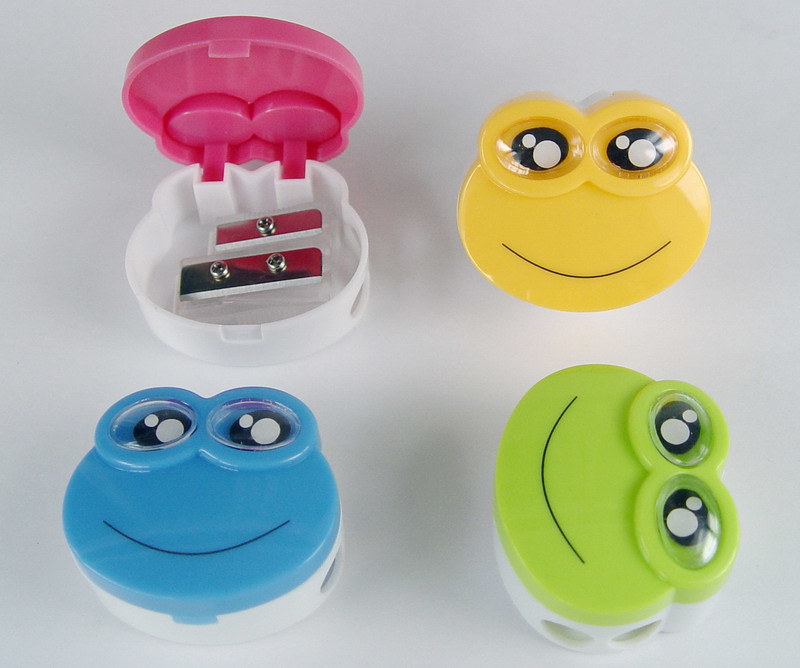The image shows a top-down view of four frog-shaped pencil sharpeners arranged on a white surface. Each sharpener features a smiling frog face with black and white eyes that protrude slightly, creating an endearing, bug-eyed appearance. The color scheme for the sharpeners includes a blue frog pointing downward, a green frog on the bottom right pointing to the left, a yellow frog also pointing downward, and a pink frog in the top left corner with its lid open. The open pink sharpener reveals its white plastic base and two angled razor blades designed for sharpening pencils of different sizes. The consistent white bases of all four sharpeners contrast with their vibrant, colorful tops, enhancing the playful and practical design of these items.